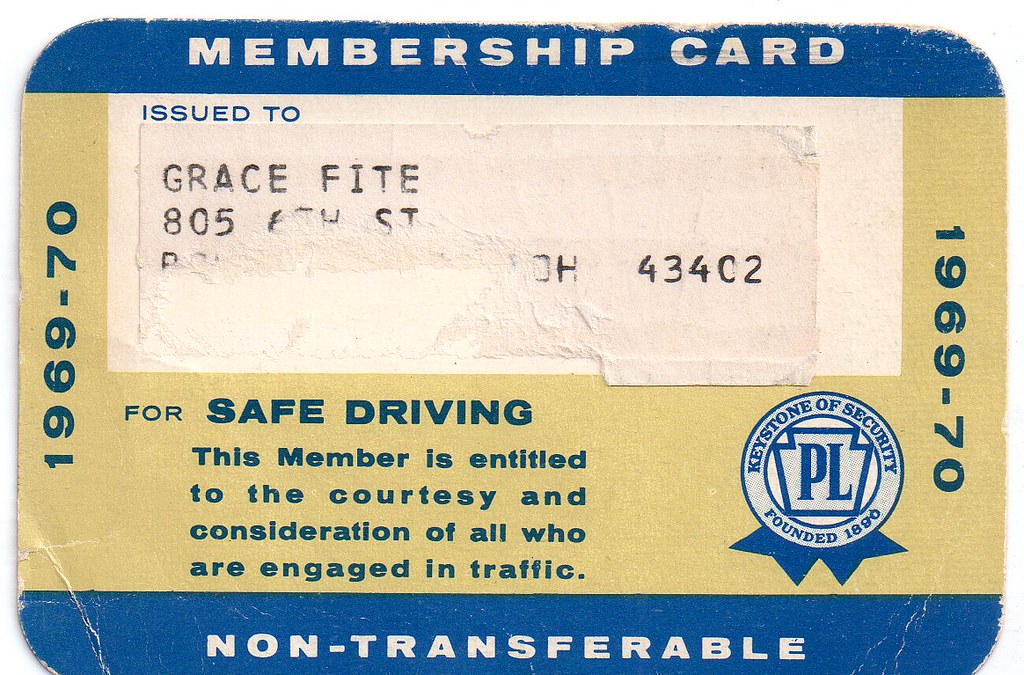This image is of a vintage membership card designed to promote safe driving and extend courtesy in traffic. The card, primarily sporting a yellowy cream background, features prominent blue bands at the top and bottom. The top band displays "Membership Card" in a cream color, while the bottom band declares "Non-transferable." 

The card is issued to Grace Fite, although part of the address, located at 805 6th Street, is rubbed out, leaving only the zip code 43402 visible, which indicates it might be from Ohio. This information appears on a white sticker in black print, situated in the center of the card.

In blue lettering along the left and right sides, it reads "1969-70," indicating the card's validity. Beneath this, it states, "For safe driving, this member is entitled to the courtesy and consideration of all who are engaged in traffic." The lower right corner holds the logo for "Keystone of Security, founded in 1890," also in blue. The overall design, including the beige-ish card color and blue accents, gives it a distinctly vintage and official appearance.